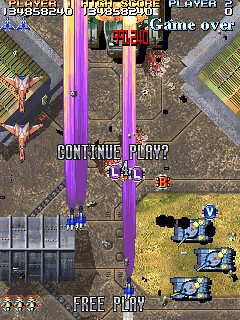A low-resolution, pixelated screenshot from a retro-style video game, reminiscent of classic consoles such as the Color Game Boy. The game operates in portrait orientation and features a war-themed setting with a bird's-eye, top-down perspective.

In the bottom right corner of the image, three blue-bodied tanks are visible, their turrets turned to reveal their guns prominently. On the left side of the screen, a couple of orange-bodied planes with white details can be seen, completing the militaristic scene.

The gameplay status indicates "Game Over" in the top right corner, suggesting the end of the current game session. The central text prompts the player with "Continue Play," while the bottom middle offers a "Free Play" option. The displayed score at the top of the screen shows the results of the game, providing a viewpoint into the player's performance and the interactive choices available moving forward.